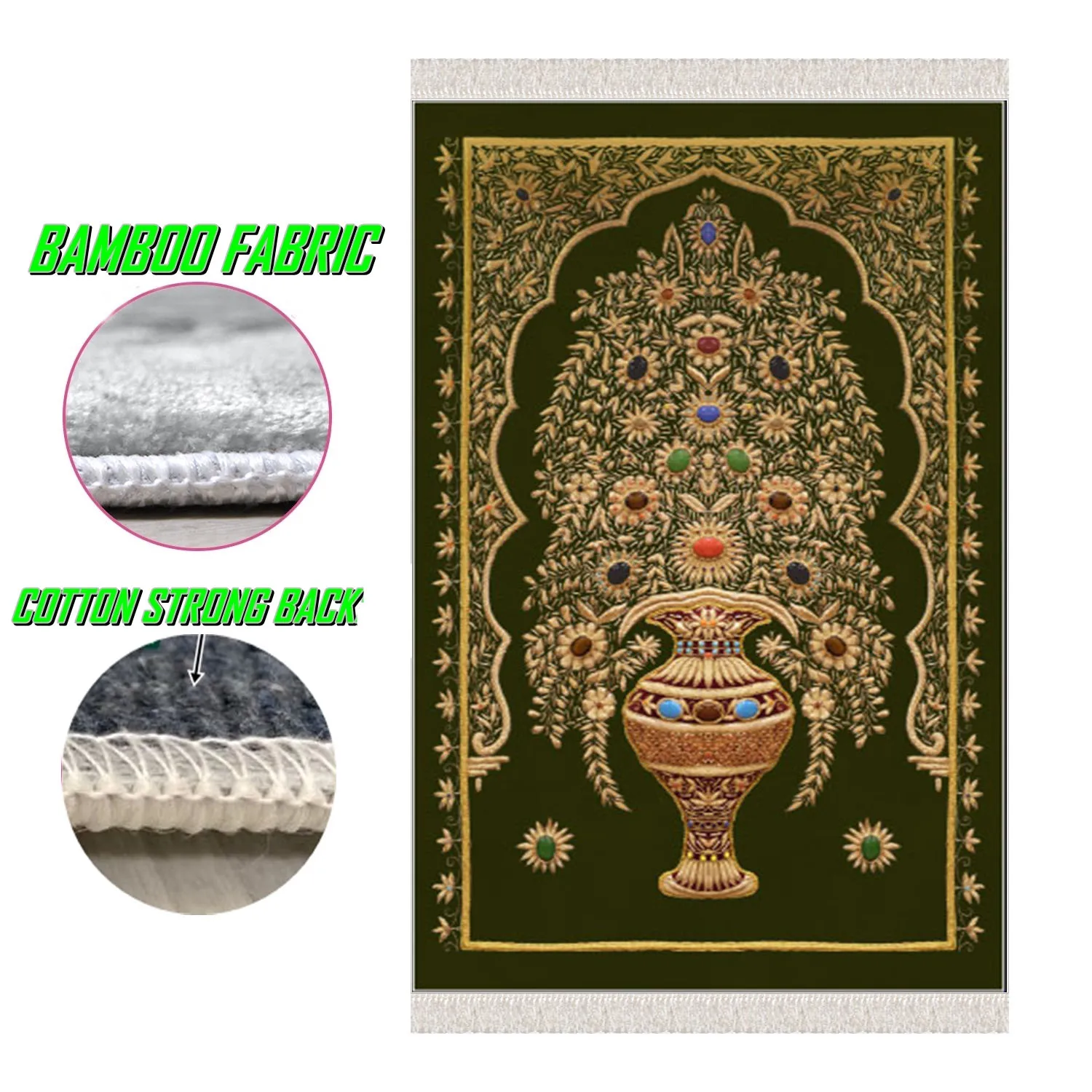This image features a detailed advertisement of an oriental-style tapestry rug with intricate designs. The rug has a green background adorned with gold detailing, featuring a central ornate vase from which golden leaves and flowers with colorful centers (red, green, blue, black) emerge. The vase is positioned towards the bottom of the rug, and the flowers, along with the leaves, create a rich tapestry embellished with an Arabic filigree pattern. The border of the rug showcases delicate golden petals and leaves.

To the left side of the rug, there are two circular insets featuring close-ups of the fabric. The top circle, outlined in dark pink, depicts a section of the edge of the tapestry and is labeled "Bamboo Fabric" in italicized, medium green, sans-serif, capitalized text. Below this, the bottom circle shows a detailed view of the rug's backing, described as "Cotton-Strung Back" in the same bright green font. The overall effect is a luxurious and meticulously crafted tapestry presented with attention to both visual and textual details.